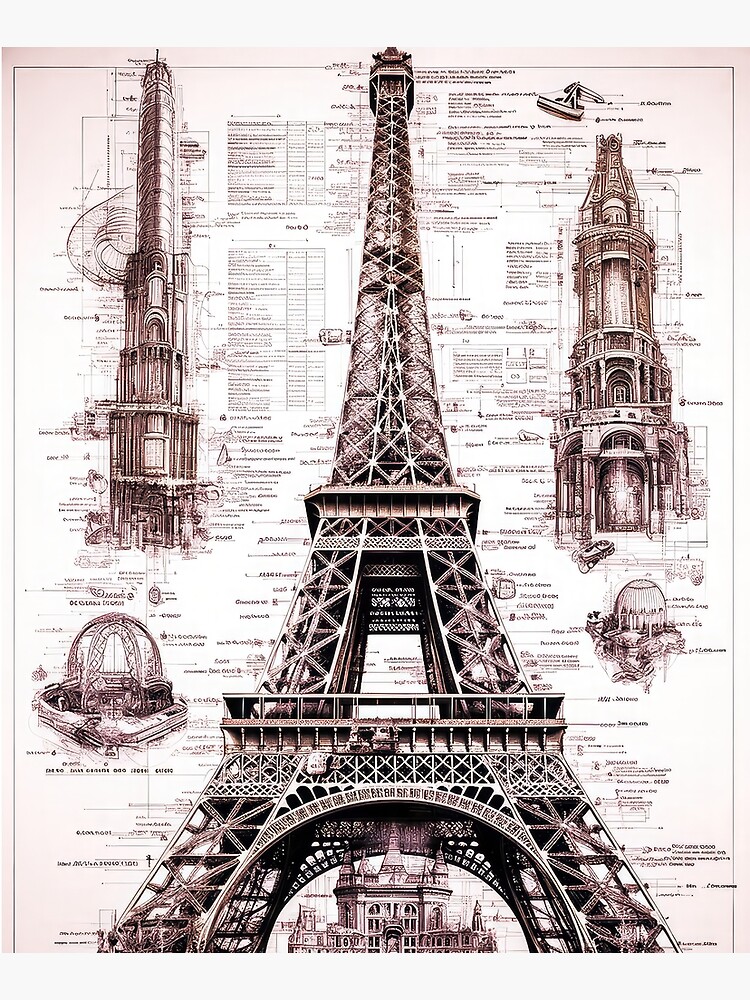This image is a highly detailed, black-and-white sheet of paper that prominently features a central diagram of the Eiffel Tower, surrounded by various smaller buildings and structures. The page is filled with intricate, tiny writing that labels different parts of these diagrams, although the text is too small to be legible. The primary focus is the intricately drawn Eiffel Tower, accompanied by what appears to be a castle at the bottom of the page and additional high-rise and circular buildings on the left and right. While the overall color scheme is black and white, some areas exhibit a subtle burgundy tint, giving the paper a faint pinkish hue against an off-white background. This art print, reminiscent of a historical design or architectural blueprint, is packed with meticulous detail, making it a fascinating piece despite the unreadable text.